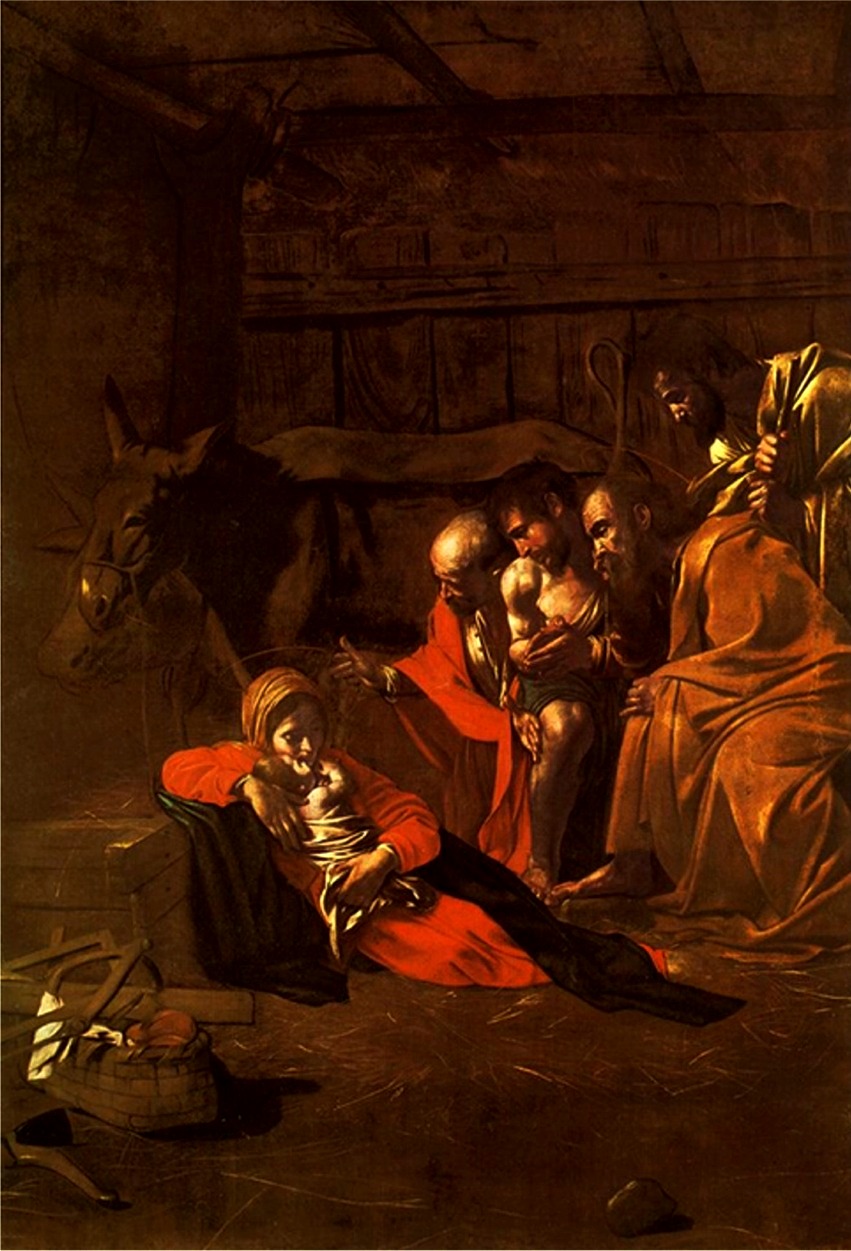This painting, reminiscent of a Rembrandt style, depicts the nativity scene within a dimly-lit manger. Dominated by hues of red and brown with strategic white highlights, the image centers on Mary, dressed in a red robe and headscarf, cradling the newborn baby Jesus swaddled in white cloth. Surrounding her, four men—potentially shepherds—are shown humbly gazing downward at the infant. One of these men is bald and garbed in a red outfit, another, a fair-skinned man with a black beard and mustache, appears shirtless. The remaining two figures are in brown robes, reverently contemplating the holy sight. A brown cow stands subtly in the background of the dark wooden manger, while faint light illuminates the soil on the left side of the scene, emphasizing the serene and sacred atmosphere.